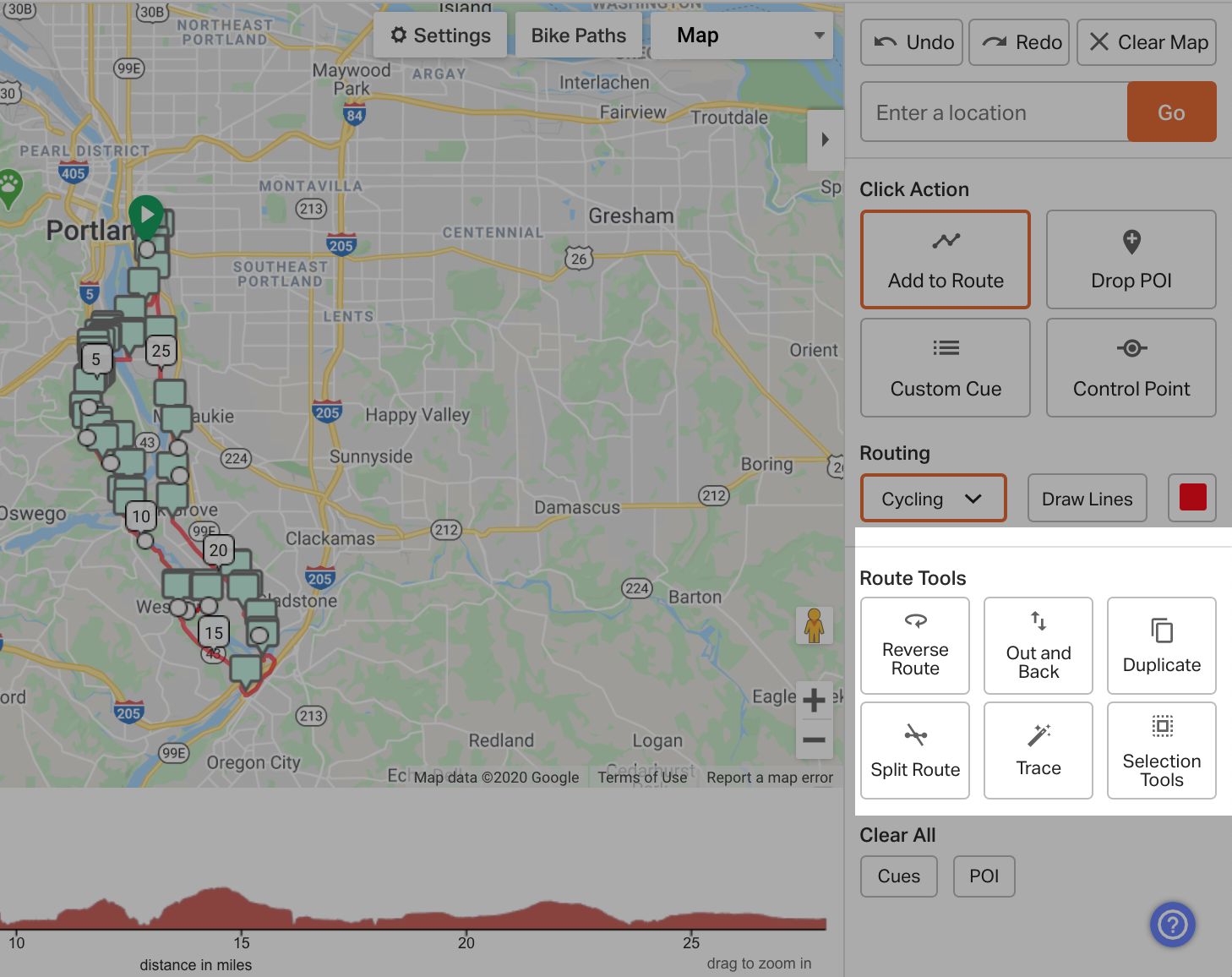The image depicts a detailed map displayed on a computer screen, centered around the Portland, Oregon area. Prominently featured is a river winding its way through the map. At the top of the screen, a settings menu is visible along with a bike path symbol. The map interface includes various interactive tools and features, such as selectable areas and clickable boxes to enhance customization options. Among the tools displayed are options for tracing routes, splitting routes, creating reverse routes, and duplicating paths. There is a selection of drawing and cycling tools, including the ability to add lines, points of interest, custom queues, and control points. A notable orange "Go" button stands out on the interface, likely for initiating an action or command. The bottom portion of the screen shows a distance metric in miles, marked at intervals of 10, 15, 20, and 25 miles, along with additional segments on the map.